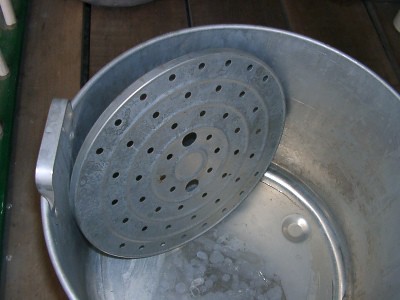This is an image providing an overhead view looking straight down into a metal bucket, potentially made of stainless steel or galvanized metal. Inside the bucket, there's a lid or circular disc featuring a series of concentric rings, each with an increasing number of holes. Notably, the middle ring has two large holes. The bucket, which has a stainless steel handle welded onto its side, is resting on a wooden surface made of brown wood slats, hinting it might be a dock or shelf. The metal piece inside the bucket has an appearance that could suggest hard water deposits. The detailed view and the overall setup suggest the bucket might be a specialized container, possibly a bait bucket, with the perforated disc designed to hold or strain contents such as fish bait.